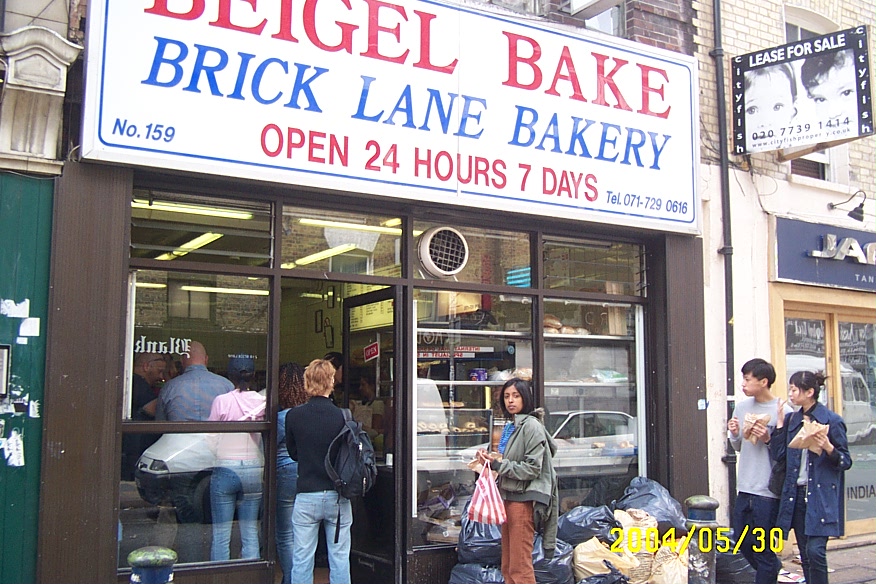This is a full-color photograph taken outdoors in a city during the daytime, dated May 30th, 2004. The image captures the bustling exterior of the Bagel Bake, Brick Lane Bakery, located at 159 Brick Lane. The bakery, identifiable by its large, white sign with "Bagel Bake" in red and "Brick Lane Bakery" in blue, is open 24 hours, 7 days a week. The sign also displays the telephone number 071-729-0616. The storefront is entirely glass, allowing a clear view of the inside where a line of customers extends out onto the sidewalk. The diverse crowd includes people holding food and walking by, as well as a couple standing in front of the bakery eating their purchases. A notable detail is the large pile of black trash bags next to the bakery. In the upper right-hand corner of the image, a "City Fish Lease for Sale" sign is visible, adding to the vibrant and somewhat cluttered city streetscape.